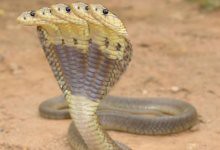The photograph captures a dramatic scene of a cobra on a plain, sandy surface scattered with a few small rocks. The snake's dark gray body stretches up elegantly into the background, while its head and iconic hooded neck rise prominently in the foreground. The cobra's underside is pale, accentuated by a dark stripe on its neck, above which sits a distinctive black spot. The image creates the illusion of the snake having three to five overlapping heads due to its rapid side-to-side movement or possibly a semi-blurred effect from the motion. The backdrop is light brown dirt with a few sporadic white spots and a hint of green in the top right corner, adding subtle contrast to the scene.